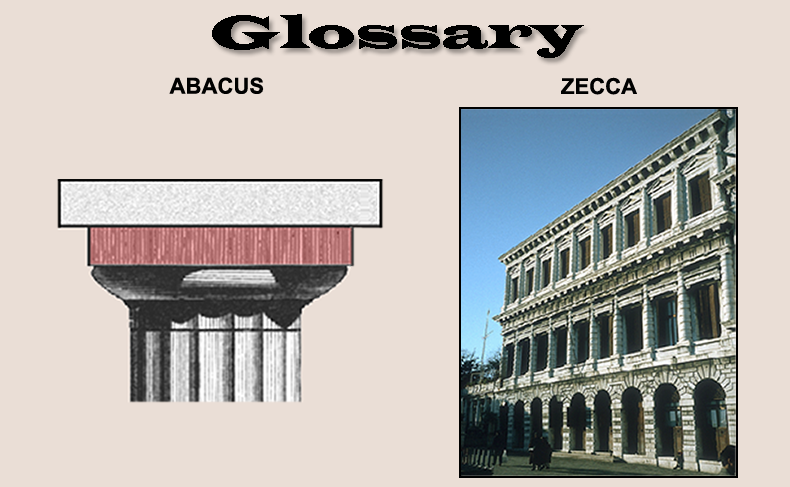The image depicts a poster in the shape of a triangle with a light, dusty pink background. At the top of the poster, the word "Glossary" is displayed in a dark or black, slightly fancy yet readable font. The poster seems to compare two subjects, labeled "Abacus" on the left and "Zecca" on the right.

On the left side, beneath the word "Abacus," there is a detailed image of the top of a classical pillar reminiscent of Roman architecture. This pillar is characterized by intricate detailing and appears to be a cropped portion of a larger photograph.

On the right side, under the word "Zecca," there is a vertical rectangular image of a three-story building featuring stone and brick architecture. This building is portrayed with several grand columns and is seen from a low angle, making it appear towering and massive. The scene includes a pale blue sky and a few blurred figures at the bottom, providing a sense of scale and depth. Sparse green grass is also visible near the base of the building.

Overall, the juxtaposition of the classical pillar on the left and the imposing building on the right suggests a comparison between different architectural styles or elements within the same thematic framework.